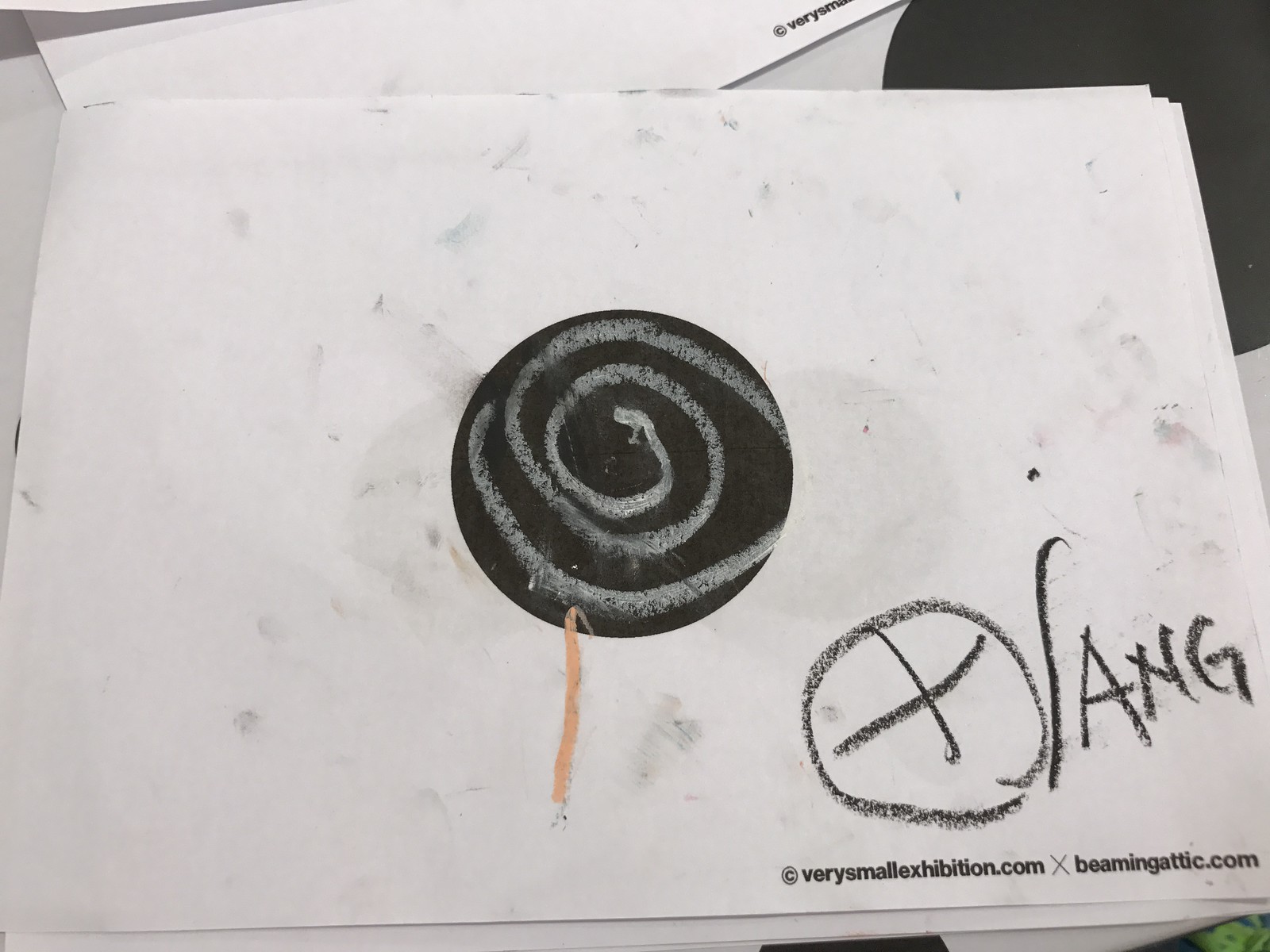The image depicts a detailed drawing on a stained, white piece of paper, showcasing a creative combination of swirling patterns and text elements. At the center of the paper lies a prominent black circle, within which a spiral pattern has been meticulously drawn using a cloudy white ink or gray pastel, creating a swirling effect that is partially filled. From the base of this black circle, a peach-colored line extends downward, resembling a lollipop stick. Towards the bottom right of the paper, there is text that reads "X/A-N-G" with the 'X' encased in a circle, all drawn in black crayon. Below this, in a small type font, is a partially visible web address or copyright notice that reads: "copyrightverysmallexhibition.com, xbeamingattic.com." The paper itself is adorned with multiple dark smudges and stains, accentuating the hand-crafted nature of the artwork.